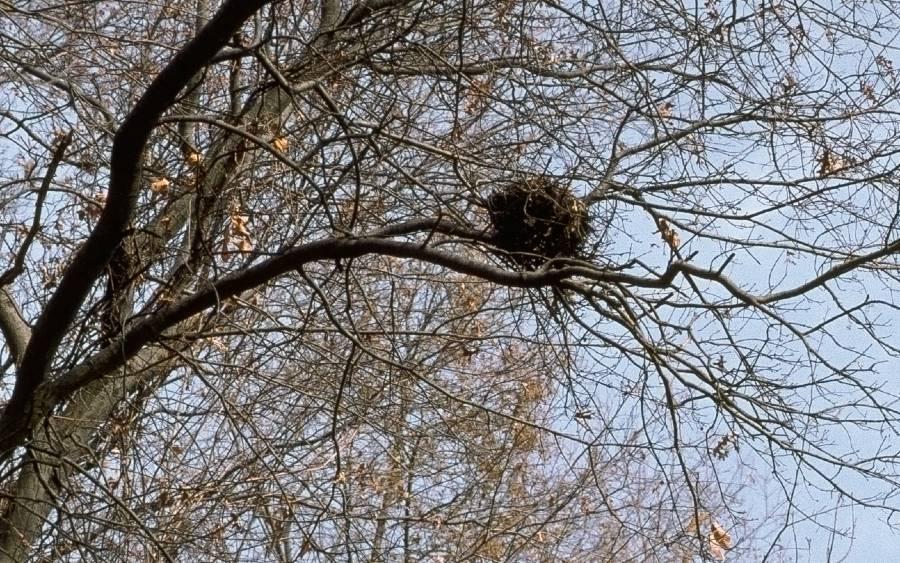The image captures a scene of a large tree canopy against a light blue sky, dominated by numerous bare branches that intersect and fan out, creating a complex web-like pattern. Sparse brown leaves are scattered throughout the branches, which are mostly thin except for two large, thick branches that originate from the bottom left corner and extend upwards into a 'Y' shape. Positioned centrally within this 'Y' formation is a prominent bird's nest made of needles and twigs, exhibiting a brown tint with a darker underside. The nest, resembling a small ball of straw, is likely the focal point of the image. The photograph, taken from a ground-up perspective, emphasizes the intricate network of twigs and branches, with the expansive sky providing a hazy blue backdrop.